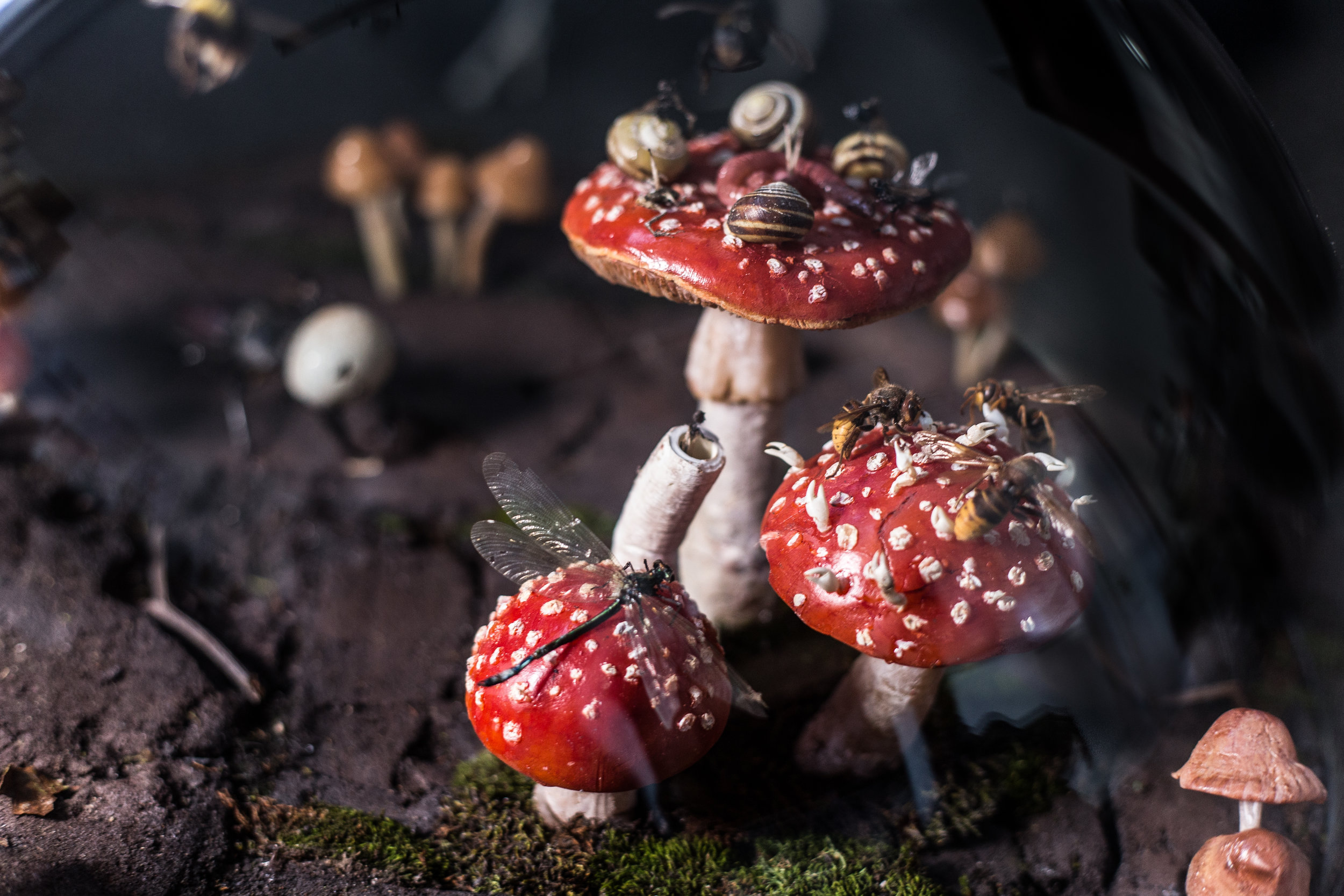The photograph showcases a detailed close-up of three red-capped mushrooms with white dots and white stems, situated on a patch of lush green moss that appears to be on soil or possibly a tree. The mushrooms are of varying heights: the smallest one is at the front, the medium-sized mushroom to its right is twice as tall, and the largest mushroom, positioned behind the other two, is twice as big as the medium one. The smallest mushroom features a dragonfly perched delicately on its cap, while the medium mushroom is adorned with several honeybees. The largest mushroom, the focal point due to its size, has four snails crawling over its cap. The background is slightly blurred, revealing an array of other mushrooms, including clusters of brown and solitary white mushrooms, as well as a couple of peachy-orange mushrooms in the bottom right corner. This assemblage of various insects and mushrooms creates a whimsical and seemingly surreal scene, raising questions about its authenticity due to its high level of detail and the unusual congregation of creatures.